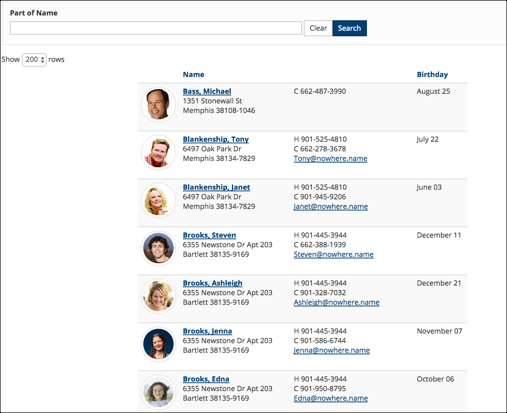The image is a screenshot of a website, outlined by a thin black border. At the very top, the header area features a light gray background with the text "Part of Name" prominently displayed in black print, with both 'P' and 'N' capitalized. Beneath this header lies a search bar.

To the right of the search bar, there's a white square button labeled "Clear" with a capital 'C'. Adjacent to it, a navy blue button marked "Search" appears, featuring white text. 

Below this, a section begins with a white background containing the word "Show," next to a drop-down menu set at '200' flanked by up and down arrows. Further to the right, the text "Rose" is followed by blue text reading "Name."

Descending into the main content area, each entry starts with a circle containing a person's image. There are a total of seven different individuals listed. Each entry details information in a structured format: last name first, followed by a comma, then their first name. This is accompanied by the person's address and phone numbers. Phone numbers are categorized as 'C' for cell phones or 'H' for house numbers, with some entries showing both types. Email addresses are also provided for some individuals, and each entry concludes with the person's birthday, displaying only the month and day without the year.